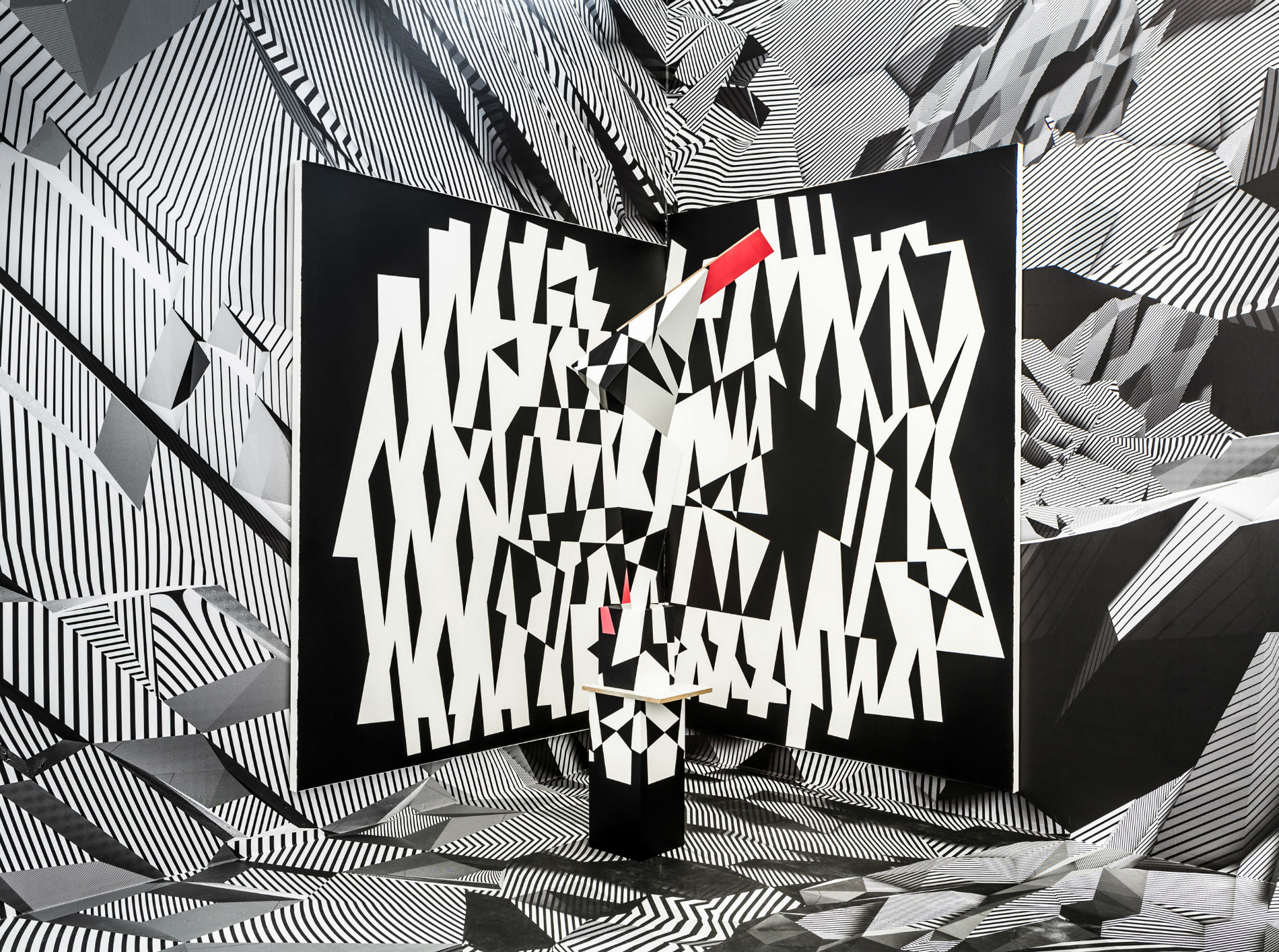This image showcases an intricate piece of abstract art dominated by black and white geometric designs. Central to the composition are two connected vertical panels forming a 90-degree angle. These panels, predominantly black with thick white lines and rectangles reminiscent of overlaying tape, also feature small red stripes, adding a subtle splash of color. The scene is further enriched by the room's op art-styled backdrop, which enhances the three-dimensional illusion with its intricate black and white patterns.

Additionally, a tall box akin to a shoebox standing on end is positioned at the base where the two panels meet, serving as a supporting structure and further displaying abstract art with similar black and white designs. Within this complex visual setup, geometric precision and sharp-edged forms prevail, creating a visually striking and immersive experience. The entire setting, with its sharp contrasts and strategic use of minimal coloring, epitomizes a harsh, op art aesthetic that challenges the viewer's perception of depth and form.